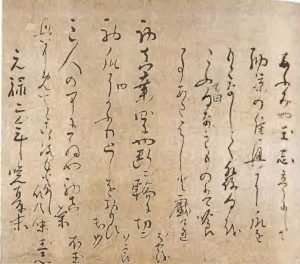The image depicts an aged piece of parchment paper, resembling an old scroll, featuring vertical lines of intricate East Asian script, likely Chinese or Japanese. The parchment has a weathered, tea-stained appearance, adding to its antique feel. The script consists of ten vertical lines of black or dark brown characters, meticulously written in straight columns from top to bottom. In addition to these primary columns, there are four distinct sections of writing at the bottom, separate from the main script. These sections contain more text, some of which are shorter, while others are longer, possibly indicating annotations or additional commentary. The overall aesthetic of the piece suggests a historical or scholarly document, rich in cultural significance.